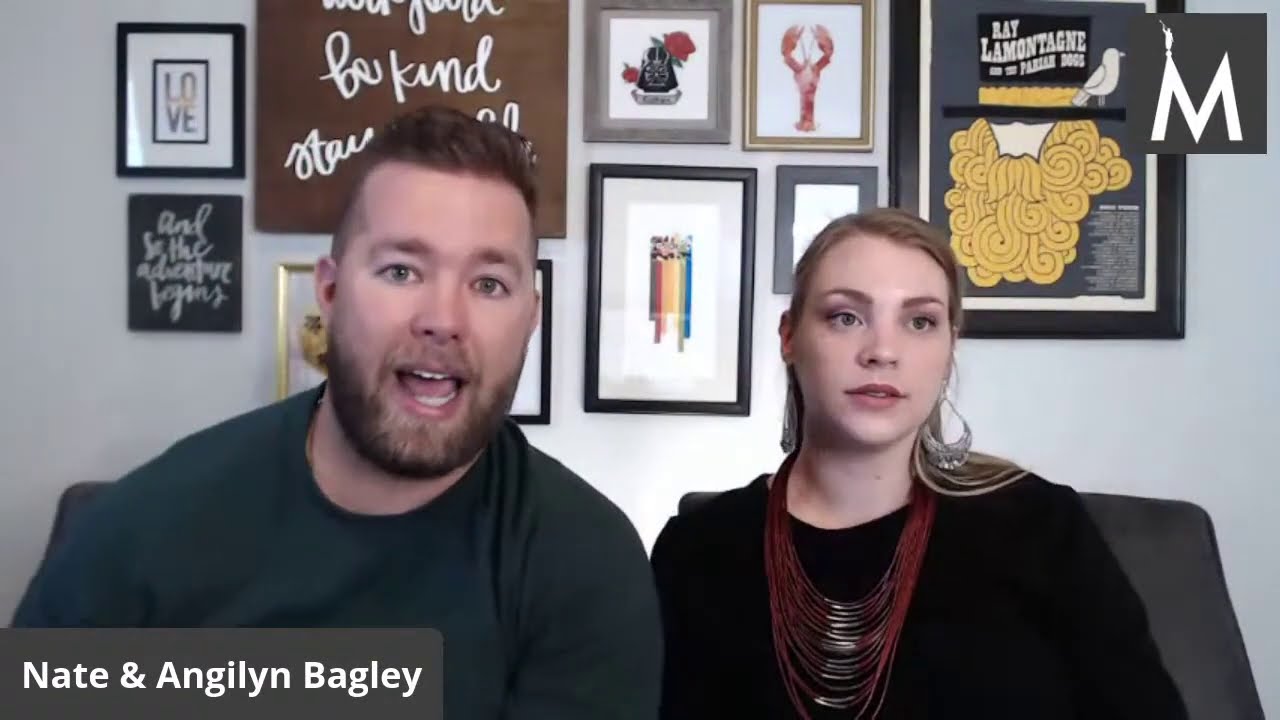The image features a Caucasian man and woman seated next to each other, visible from the torso up. The man, on the left, has short brown hair, a mustache, and a beard with blue eyes. His mouth is open, revealing his tongue and rows of teeth. He is dressed in a long-sleeved dark gray or blue shirt. The woman to his right has dark blonde, straight hair that reaches her shoulders with a left-side swoop. She has brown eyes and is adorned with very long silver earrings and a multi-strand necklace draping across her chest, which appears red in color. She wears a long-sleeved black shirt. 

They are sitting on a gray chair or couch. The background wall is decorated with various framed pictures, including ones with a crab, the word "love" in two lines, and a man with a large golden beard and a top hat with the text "Raylon Montage" and a bird illustration. In the bottom left corner of the image is a gray square with white text reading "Nate and Angeline Bagley."